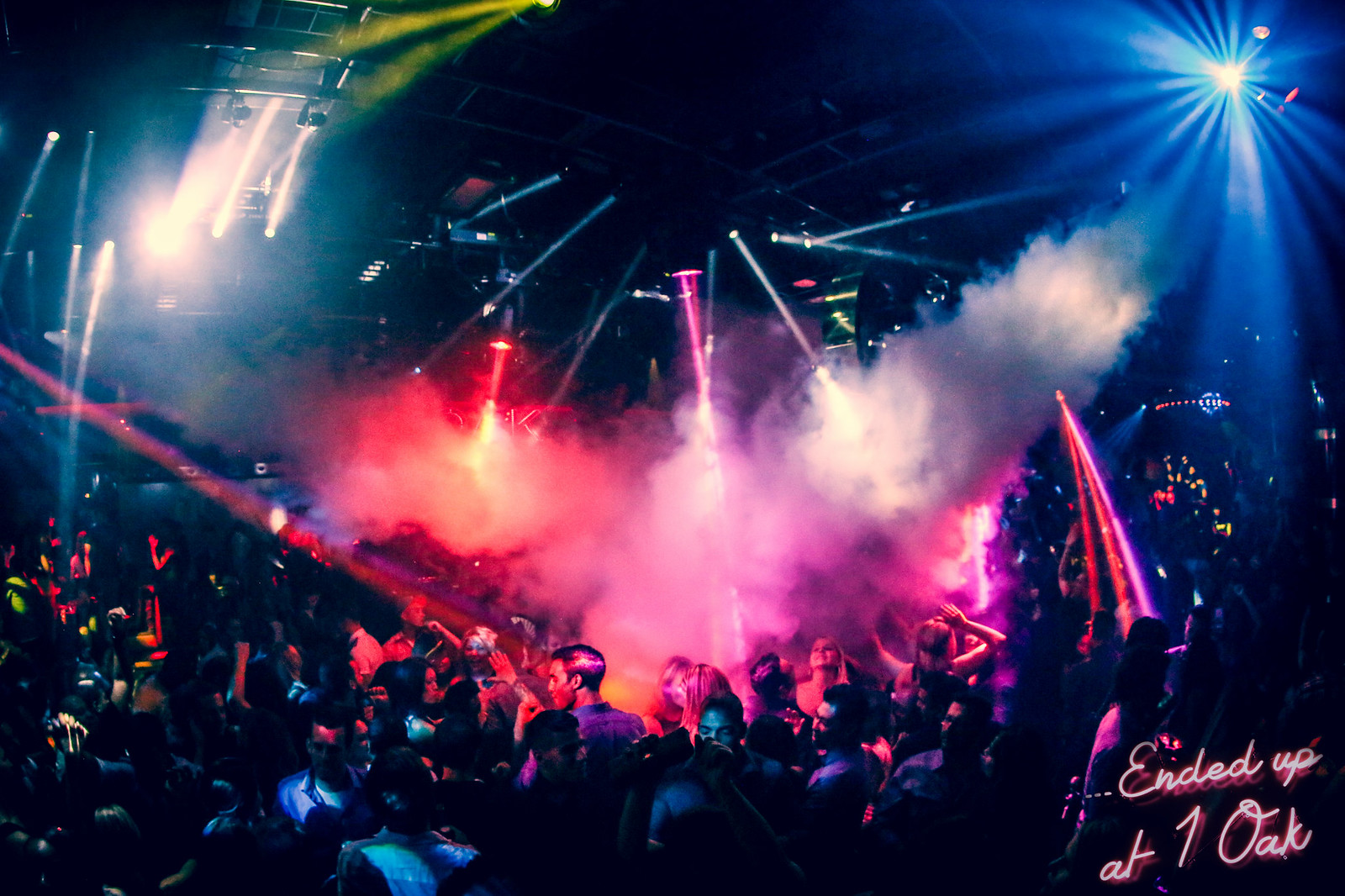The image portrays a vibrant nightclub scene, likely at a concert or dance event, filled with a large, bustling crowd of men and women. The atmosphere is dark, but the scene is brought to life by an array of vivid lights in reds, blues, oranges, pinks, and purples, which pierce through clouds of pink, white, and purple smoke billowing from the left side. Overhead, sweeping beams of white light glance off the shoulders and faces of the attendees, creating a dynamic, almost ethereal effect. The crowd is densely packed on the dance floor, with people dancing and their hands raised, moving around in seemingly all directions. Notably, in the bottom right corner of the image, there is a handwritten-style text that reads, "Ended up at One Oak."